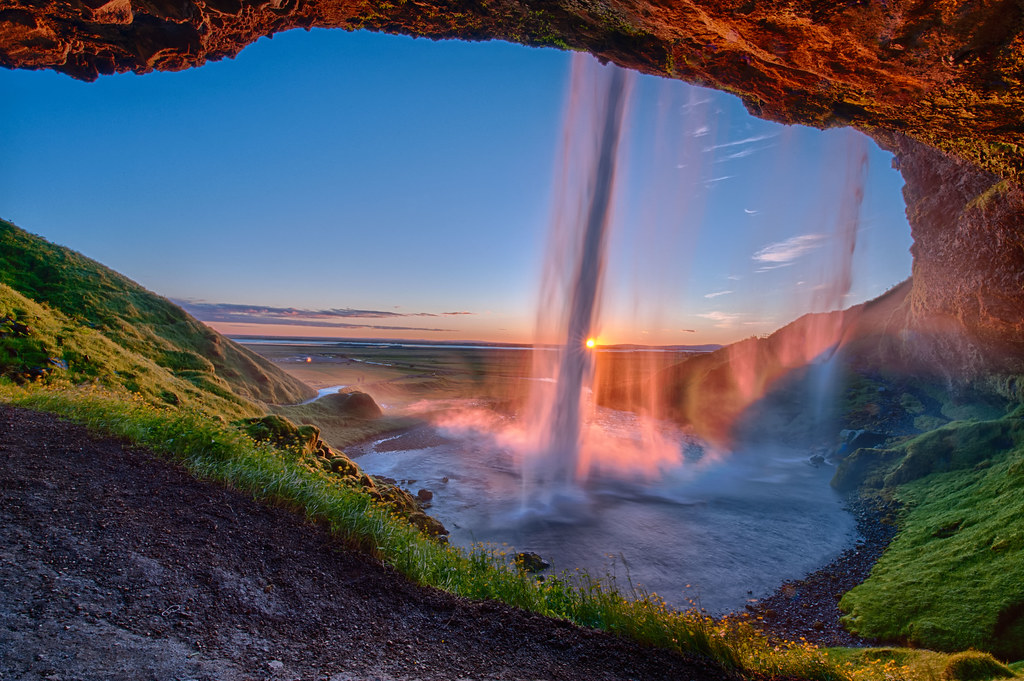Under a vibrant blue sky, an impressive geological formation with an orange-hued stone top stands prominently. At its peak, a waterfall cascades down, contributing to a larger water flow that descends into a serene lake below. The falling water disperses widely as it reaches the lake, creating a dynamic and refreshing scene. Off in the distance, scattered clouds dot the sky, with the sun faintly visible, adding a soft glow to the landscape. On the far right, patches of short, green grass contrast beautifully with the earthy tones, while to the far left, glimpses of exposed dirt can be seen, adding a rustic touch to the natural tableau.